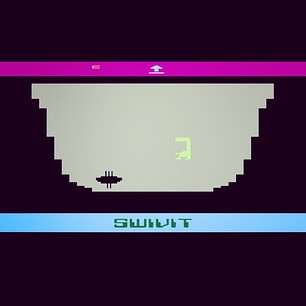A screenshot of a video game interface predominantly features a black background. A pink horizontal stripe stretches across the screen, positioned approximately one-third from the top. Within the center of this stripe is a small, upward-pointing white arrow accompanied by a line beneath it and a short horizontal line at the base. 

Directly below this pink stripe is a gray, U-shaped graphic. Nestled in the bottom left section of the U shape is a tiny bug-like figure. In the middle-right segment of the U shape appears a small green dinosaur-like character. At the bottom of the screen, a thin blue line spans across, with a green word inscribed in its center.